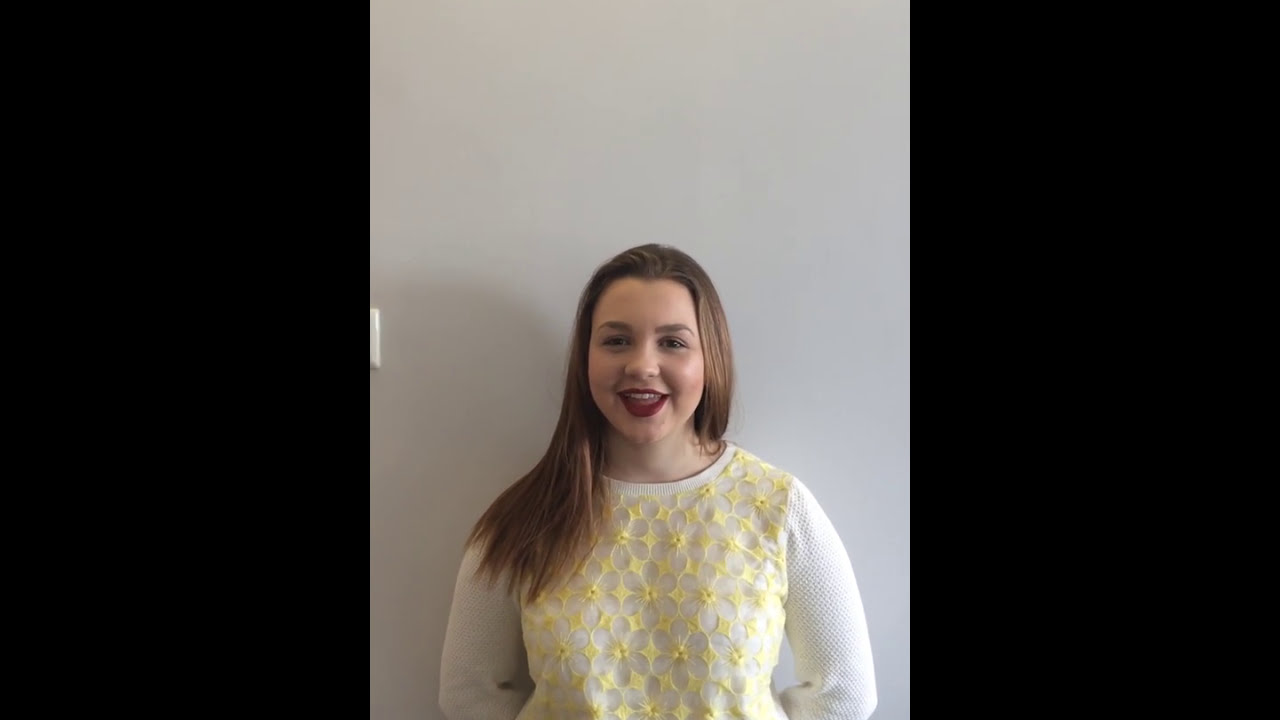The photo features a young woman standing against a plain white wall, with the faint outline of a light switch visible on the left-hand side of the image. She has light brown, or dark blonde, hair that extends slightly past her shoulders. On her left (our right), her hair is tucked behind her, resting on her back, while on her right (our left), her hair drapes forward over her shoulder. She has fair skin and is wearing red or burgundy lipstick. Her facial expression is ambiguous, with some describing it as a pouty face, while others perceive it as a smile. She is dressed in a white crewneck sweater or shirt, adorned with a gold or yellow pattern on the front, resembling four-pointed stars or flower petals connected in a web-like design. Her arms are positioned behind her back. The photo captures her from the head down to about her midriff, with her head centered in the frame.